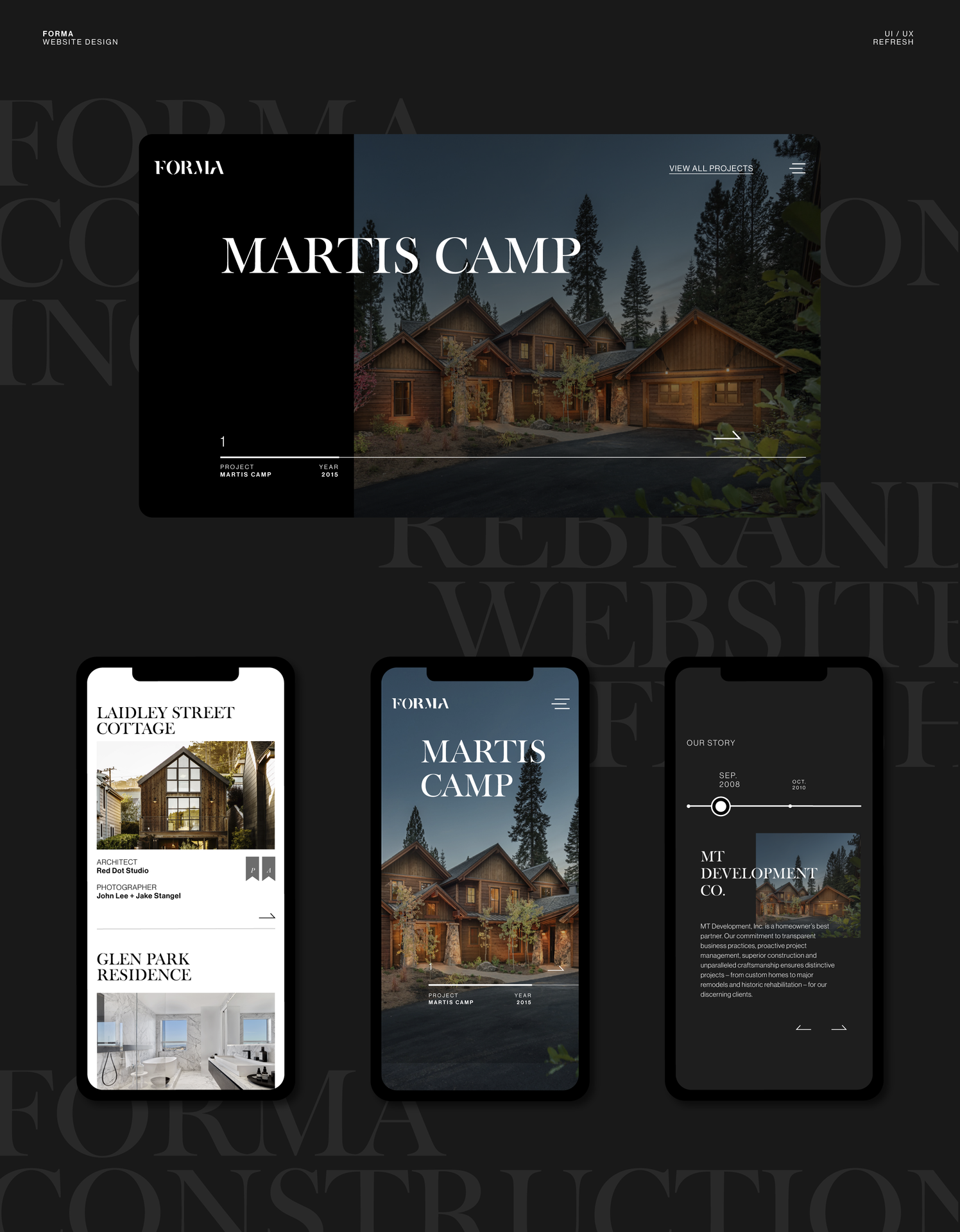This image appears to be a polished screenshot from a template website design, showcasing a refined and user-friendly layout. The background is a muted gray, adorned with lighter gray serif fonts that provide an elegant touch. The upper left corner features the title "Forma Website Design and UI UX Refresh," lending clarity to the content's purpose.

At the very top, there's a prominent image of a website project highlighted. It depicts a scene labeled "Forma" on the left and "Martus Camp" on the right. This image showcases a picturesque log cabin nestled among pine trees, complete with a driveway and a two-car garage. The image is slightly darkened, enhancing the text "View All Projects" prominently visible on it. Near the bottom center of the image, an annotated underline with the numeral "1" indicates it’s the first project, captioned "Project Martus Camp Year 2015."

Below this main header, three smartphone screenshots are presented in a row:
1. **Left:** The first smartphone displays "Lately Street Cottage," featuring another charming rustic home. The detailed description includes the architect "Red Dot Studio" and photographers "John Lee plus Jake Stangle." Bookmark icons suggest sharing options, possibly for Pinterest. 
2. **Middle:** The central smartphone showcases a responsive design adaptation of the "Forma Martus Camp" project. The truncated image centers on the cabin's facade, labeled with the project's name and the year at the top, effectively demonstrating the site's mobile-friendly layout.
3. **Right:** The rightmost screenshot is focused on "MT Development Co." with the text "Our Story, September 2008," hinting at a timeline feature. It again shows an image of the cabin and mentions "MT Development Co." with some additional details that are not legible, all set against a medium gray background.

Finally, below this segment, there's a smaller image captioned "Glen Park Residence," showcasing an interior view of a predominantly white bathroom, completing the elegant and coherent design layout depicted in this screenshot.